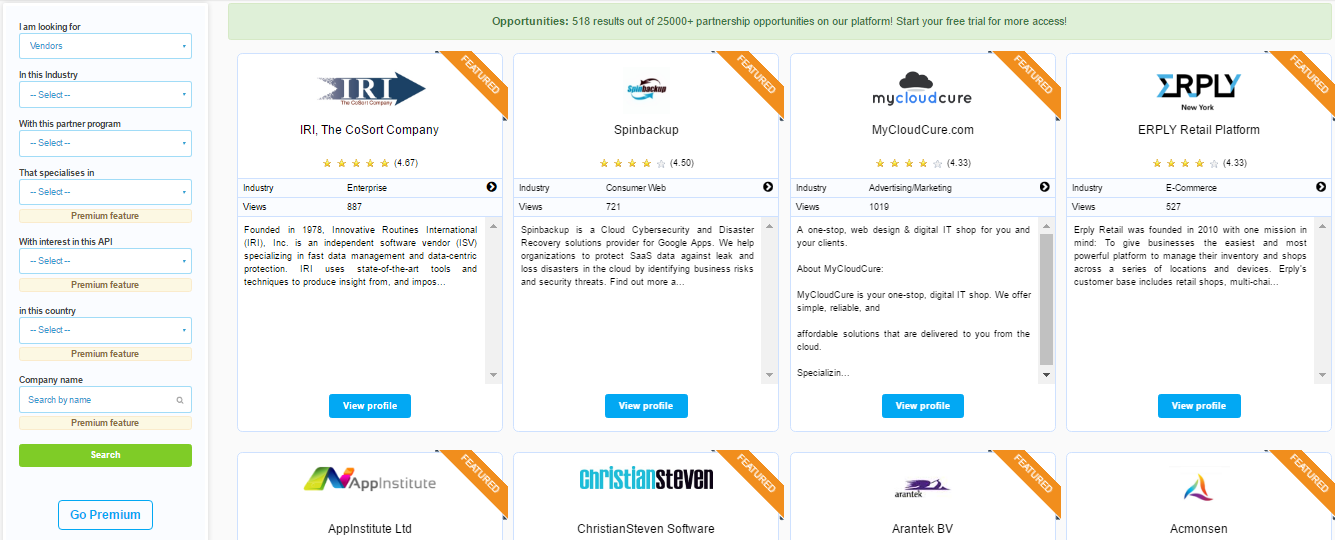In the image, a user interface is displayed featuring a column with multiple drop-down menus for selecting various program parameters. The user is expected to select options from these menus, such as choosing a specialization, enabling premium features with an interest in CPI, and selecting the relevant country and company name. There is a prominent green search bar for initiating the search, labeled "Go Premium." To the right, the interface reveals that there are 518 out of more than 25,000 partnership opportunities available on their platform. Users are encouraged to start a free trial for more access, guided by a blue arrow pointing towards the option.

The focus then shifts to details about a company named "Texas RIRI," identified as the IRI, a co-start company with a white star rating of six out of seven. This company operates in the enterprise industry, was founded in 1978, and functions as an independent software vendor specializing in fast data management and data protection using state-of-the-art tools. It offers a disaster recovery solution named "Spin Backouts," designed to help organizations protect and extend the appeal of their IT infrastructure.

Additionally, there is a mention of "Mic Cloud Care" (miccloudcare.com), which emphasizes their commitment to designing digital IT shops, particularly targeting low to middle-income youth. The platform is branded as "My Cloud Care," offering a forward-thinking survival system from the cloud.